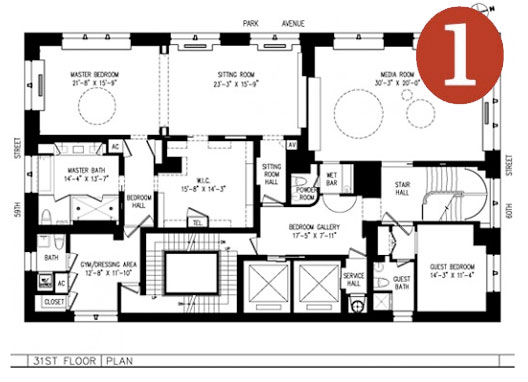The image displays a detailed floor plan of the 31st floor of a building located at the intersection of Park Avenue and 39th Street. The layout is meticulously illustrated and includes the following key features:

- **Master Bedroom (Top Left Corner)**: Dimensions are approximately 21 feet by 8 feet and 15 feet by 9 feet.
- **Sitting Room (Next to Master Bedroom)**: Measures about 23 feet by 3 feet and 15 feet by 9 feet.
- **Media Room (To the Right of Sitting Room)**: Appears to be around 30 feet by 3 feet and another dimension that is unclear but likely similar.

In the top right corner, a significant marker is present, a large red circle labeled "1."

Below the master bedroom:
- **Master Bath**: Located directly below.
- **Bedroom Hall**: Connects the master bath to a dressing area and a gym.
- **Dressing Area and Gym**: Adjoining rooms that include a bath, AC unit, and a closet.

Off of the sitting room, the following features are noted:
- **Walk-In Closet**: Located adjacent to the sitting room.

The floor plan also includes:
- **Sitting Room Hall**: Extends from the sitting room.
- **Powder Room**: Inaccessible directly from the sitting room.
- **Wet Bar**: Positioned near the stair hall.
- **Stair Hall**: Connects to the media room.
- **Bedroom Gallery**: Attached to both the stair hall and the wet bar.
- **Service Hall**: Linked to the bedroom gallery.
- **Guest Bath and Guest Bedroom**: Situated off the stair hall.

Each area is delineated with precise measurements, enhancing the functionality and accessibility of the floor layout.